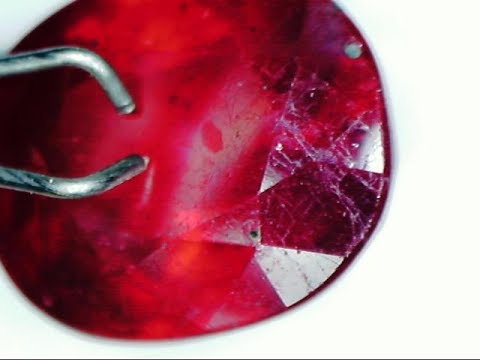This image features a close-up view of a gemstone that exhibits a deep purplish-red hue, potentially suggesting it could be a ruby or another similar precious stone. The gem has a polished finish with visible light reflections, indicating multiple faceted cuts. Its shape is generally round but irregular, and it possesses a small hole near the top, implying it could be used as a pendant. Resting on a white backdrop, the gemstone appears significantly enlarged, potentially a result of the image being cropped and magnified. On the left side of the gem, a pair of thin metal prongs, possibly from a pair of steel forceps, are positioned such that they look ready to grip the stone but are not yet making a firm hold. A thin black line runs horizontally across the bottom of the image, likely a remnant from the cropping process.